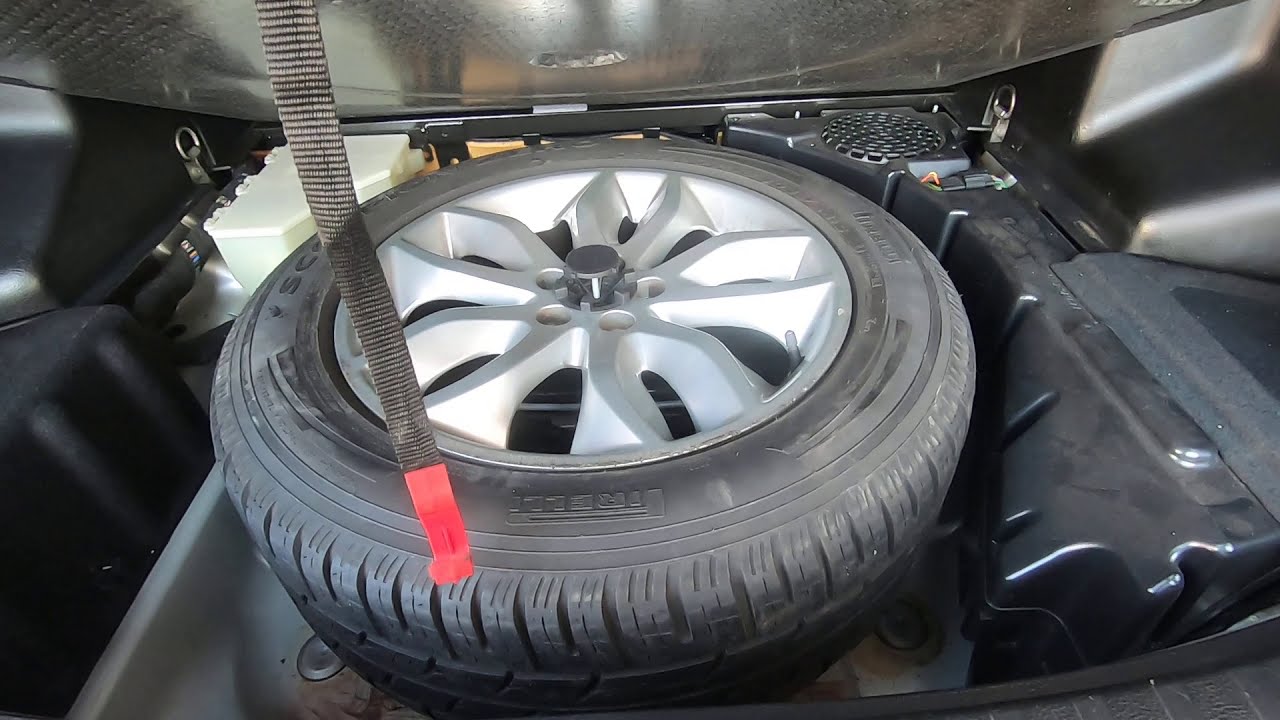This detailed photograph captures the interior of a car's trunk, specifically focusing on the spare tire storage compartment. The main feature is the spare tire with new tread, lying flat and securely bolted in place within a custom-shaped black container. The tire has a silver rim and some indistinguishable lettering on it. Above the tire, the shiny trunk floor is slightly reflective. At the top left, a black strap with a red handle hangs down close to the tire, suggesting its use in opening and closing the lid of the compartment. To the right of the compartment, various car connectors and plugins are visible, and in the back left corner, there's a boxy white object. The overall scene highlights the organized and utilitarian design of the car's trunk, with the spare tire as its central element.